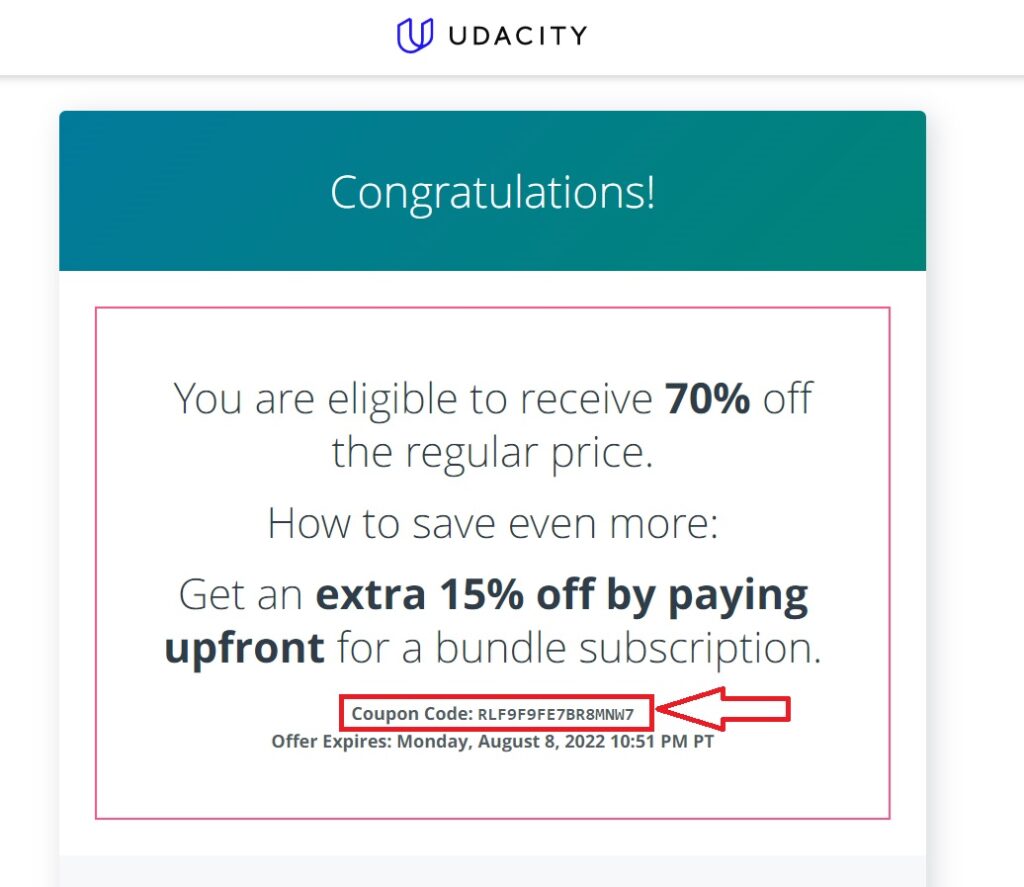The image is a screenshot from a promotional pop-up on Udacity's website. At the top, there is a Udacity logo, consisting of the text "Udacity" alongside a stylized letter "U." The background is teal, and features a bold "Congratulations!" heading in white font. Below the header, there is a prominent white rectangle outlined in red that contains the main message. The message states, "You are eligible to receive 70% off the regular price," with "70%" highlighted in bold black text for emphasis. 

Further down, the message offers additional savings: "Get an extra 15% off by paying upfront for a bundle subscription," with "extra 15% off" also in bold. In the same rectangle, there is another red-outlined section containing a coupon code comprised of uppercase letters and numbers. The offer details, "Offer expires: Monday, August 8, 2022, at 10:51 p.m. P.T.," are listed just below the coupon code.

Finally, there is a red-outlined white arrow pointing towards the coupon code, drawing attention to it. This arrow, like other elements, is designed to stand out and guide the viewer to the most critical information.

Overall, the design uses a combination of bold text, red outlines, and strategic arrows to highlight key details and enhance readability.